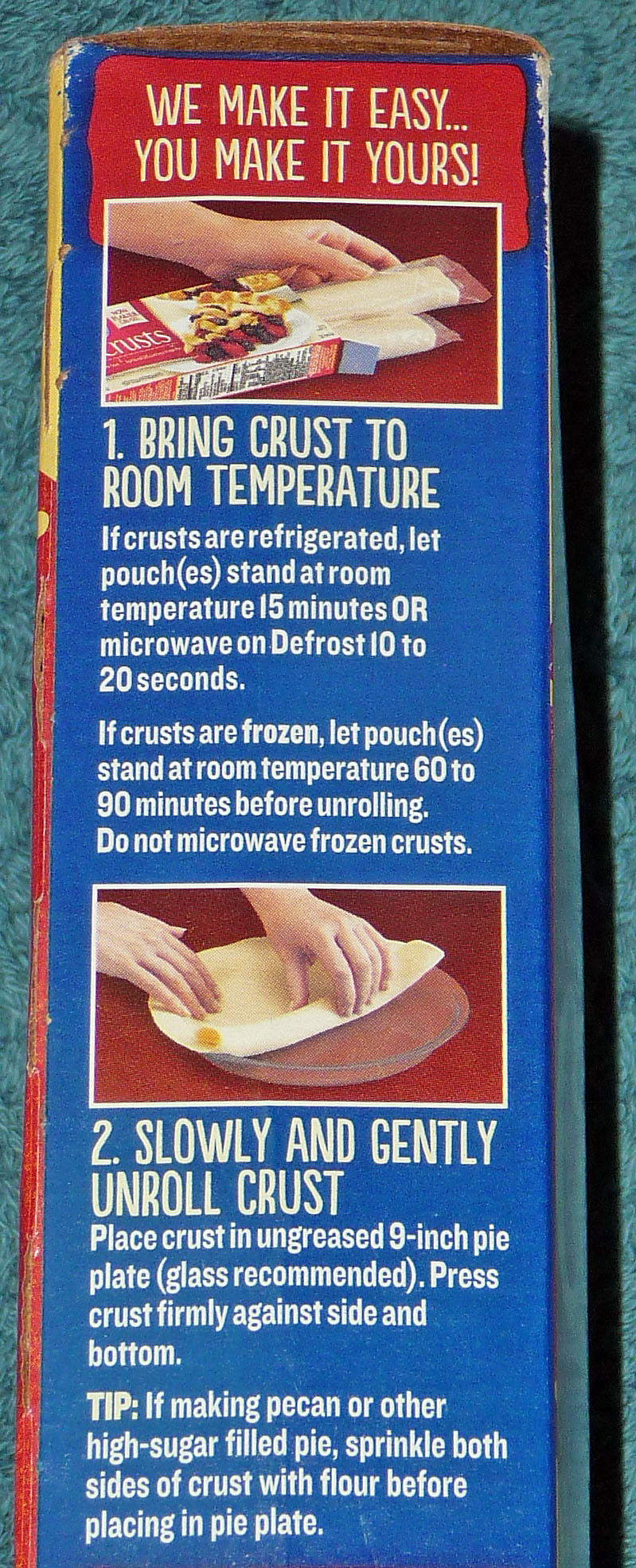This color photograph shows detailed instructions on how to prepare a pre-made pie crust, displayed on the side of the packaging. The packaging sits on a teal shag-style carpet. At the top, a red banner with white text reads, "We make it easy, you make it yours." Below the banner, there's an inset image of a woman's left hand pulling a wrapped pie crust out of a red and white box that depicts a finished pie along with a list of ingredients. In cobalt blue underneath, step one in white font instructs: "Bring crust to room temperature. If crusts are refrigerated, let pouches stand at room temperature for 15 minutes or microwave on defrost for 10 to 20 seconds. If crusts are frozen, let pouches stand at room temperature for 60 to 90 minutes before unrolling. Do not microwave frozen crusts."

Another image shows a person unraveling the crust on a plate with their hands. Further instructions in large white font state, "Step two: slowly and gently unroll crust. Place crust in ungreased 9-inch pie plate (glass recommended). Press crust firmly against side and bottom." A tip in smaller white font advises, "If making pecan or other high sugar-filled pie, sprinkle both sides of the crust with flour before placing it in the pie plate." The clear, step-by-step visual and textual guidance is meant to simplify the process of preparing the pie crust.